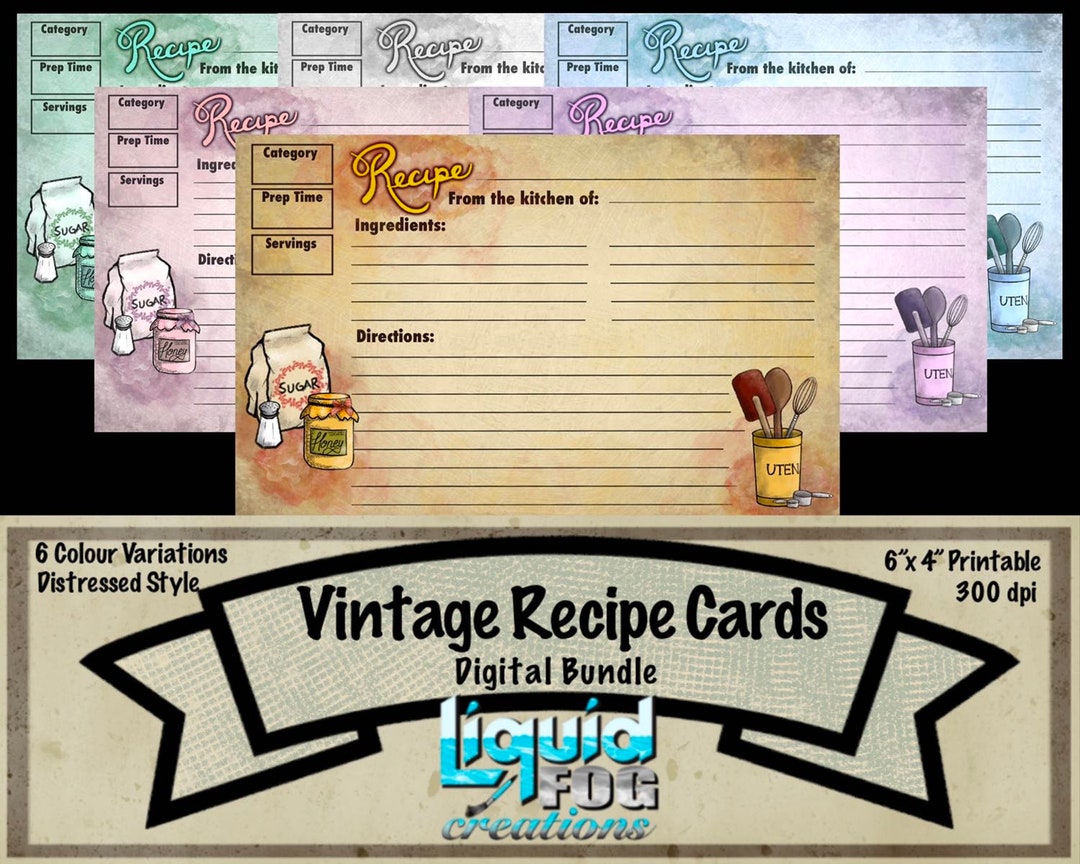This promotional image showcases a digital bundle of vintage recipe cards, each adorned with a distressed style. The upper portion of the image features six recipe cards in varying colors: light green, pink, white, darker violet, light blue, and light brown. These cards share a common template, displaying a small icon of a utensil bucket with a spatula, spoon, and whisk, and images of a salt shaker, honey jar, and sugar bag in the bottom left corner. The upper left-hand corner of each card includes labels for category, prep time, and servings. Below that, space is provided to write the recipe, ingredients, and directions. The bottom of the image details that this is a “Vintage Recipe Cards Digital Bundle” by "Liquid Fog Creations," offering six color variants, printable at 6x4 inches and 300 DPI.